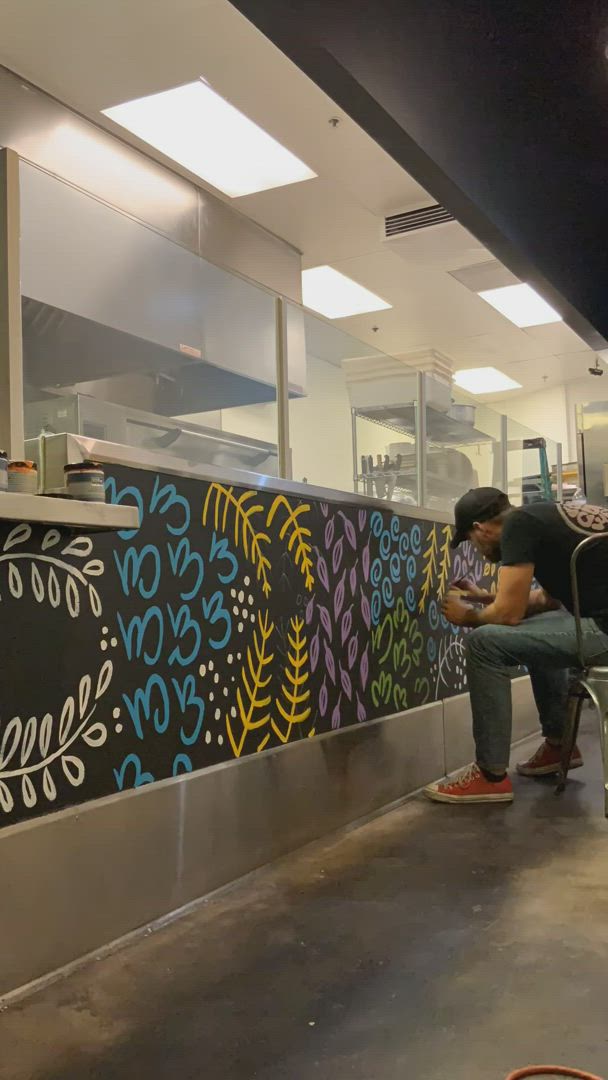In this photograph taken inside a restaurant, we observe a somewhat worn, gray concrete floor typical of an urban setting. Dominating the right side of the image is a young man dressed in a black t-shirt with a logo on the back, blue jeans, red Converse shoes, and a black baseball cap. He appears to be looking down at his phone, possibly waiting for his food.

In front of him stands a distinctive half wall that extends to about five feet in height and is trimmed with stainless steel. The wall is adorned with a vibrant mural displaying an array of colorful patterns including white, yellow, and purple leaves, blue number threes, and squiggly blue lines, all set against a black background, creating a striking, artsy atmosphere. Above the half wall, a clear glass partition allows a view into the bustling restaurant kitchen.

The kitchen, visible behind the partition, features stainless steel ovens, hoods, and other typical restaurant equipment, indicating this is an active food preparation area. To the left side of the image, a counter or shelf area, likely a pass-through, is partially seen, suggesting a place where orders are picked up. Illuminating the room are square fluorescent lights affixed to the ceiling, enhancing the environment's utilitarian yet vibrant ambiance.